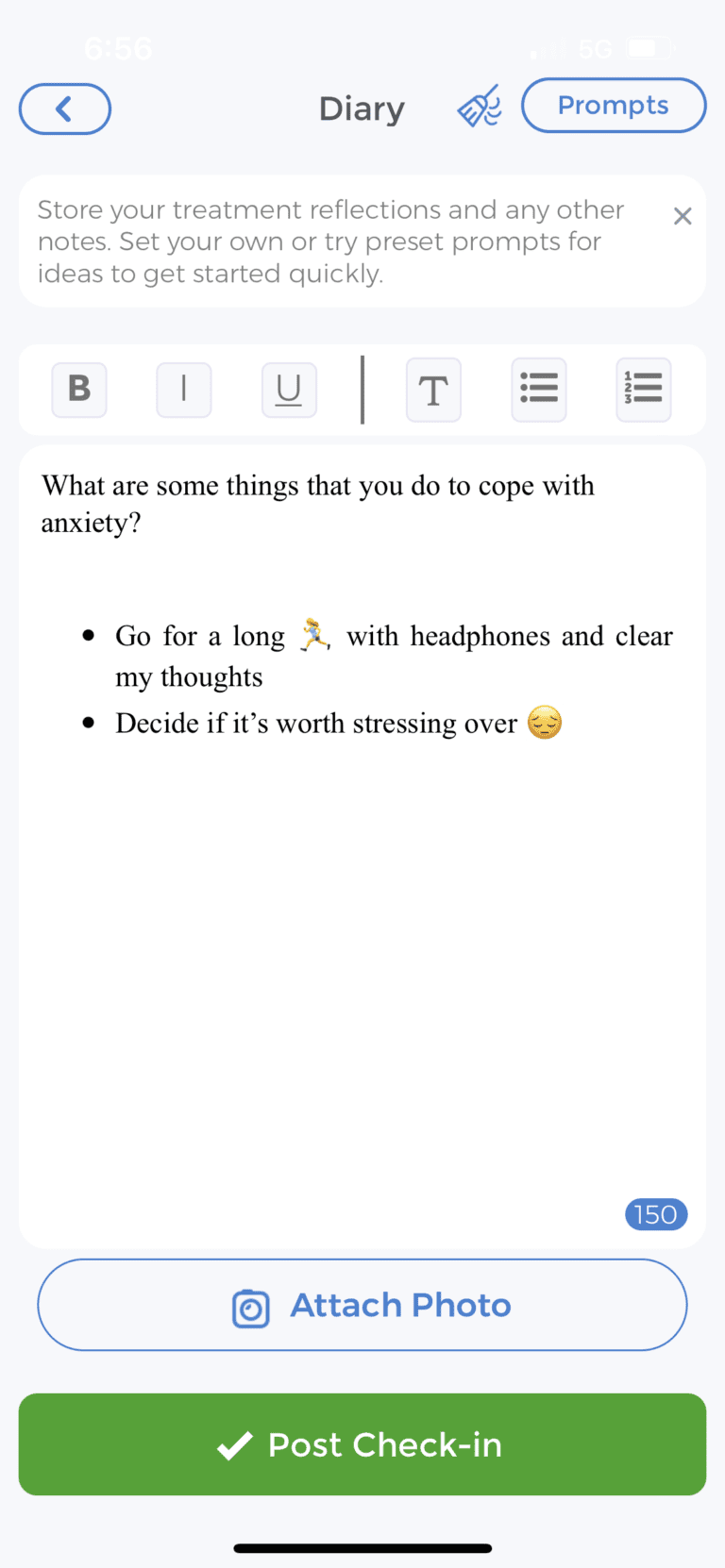Screenshot of a Mobile App - "Diary" Feature:

The screenshot displays the "Diary" section of a mobile app. At the top center of the screen, the word "Diary" is prominently visible. To its right, there's an icon resembling a broom, and immediately next to it, the word "Prompts" is written. Above this, the number "656" is displayed in white font on a gray background. The status bar at the top reveals a 5G internet connection, but the battery percentage is partially obscured. On the left side of "Diary", there's a left-facing back button.

Below the "Diary" header, a section with a white background contains the text: "Store your treatment reflections and any other notes. Set your own or try preset prompts for ideas to get started quickly."

Further down, various formatting options are visible:
- A bold button logo.
- An italicize button to its right.
- An underline button following that.
- A dividing line separates these from a "T" logo, likely for font styles.
- Options for adding bullet points and numbered lists are also present.

Under these formatting tools, a prompt reads: "What are some things that you do to cope with anxiety?" followed by two bullet points:
1. "I go for a long walk or jog." Accompanied by an icon of a lady jogging with headphones.
2. "I decide if it's worth stressing over." Accompanied by an emoji depicting a gloomy or depressed face.

Towards the bottom right of the section, a word or letter limit of "150" is indicated. Below, there is an option to attach a photo and a green button labeled "Post Check-in".